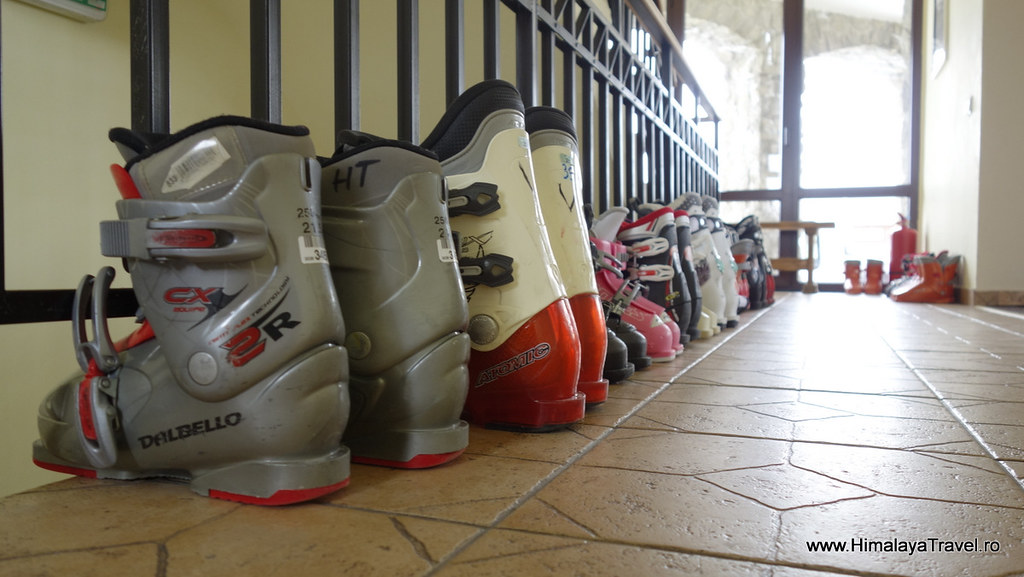The photograph showcases a dramatic, low-angle view of numerous ski boots of varying shapes, sizes, and colors, neatly propped up against a black wrought iron railing on the left side of the image. The boots are arranged on a distinctive brown tile floor with a diamond-shaped pattern in the middle of the tiles, extending into the distance. The boots range from larger sizes on the left, such as a gray pair with red accents and the brand name 'Dalbello' displayed prominently, to smaller sizes that gradually disappear towards the middle right of the frame. The boots exhibit a mix of hues including gray, red, black, white, and pink, and appear to be made of hard plastic materials. There are also some rain boots situated to the right of the ski boots. A large glass window with a black frame and a brick awning is visible in the background, casting natural light into the scene. On the bottom right corner of the image, a website URL, www.himalayatravel.ro, is displayed, indicating perhaps a connection to a travel or rental business. The overall scene suggests a setting where these used boots are possibly waiting to be rented out or sold, similar to a thrift store.